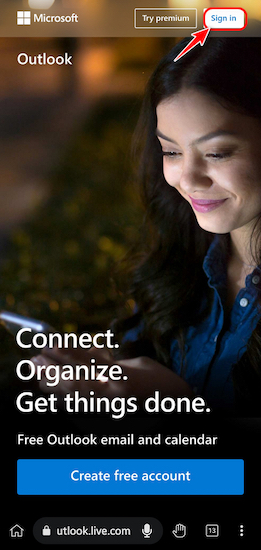This promotional image prominently displays a Microsoft Outlook web page. At the top left corner, the Microsoft logo is clearly shown. In the top right corner, options to "Try Premium" and "Sign In" are available, with a red arrow emphasizing the "Sign In" button. The main content features a background image of a woman using a mobile device in a dimly lit setting, reinforcing the idea of staying connected anywhere. Inspirational text reads "Connect, organize, get things done," followed by the offer for "Free Outlook email and calendar." Users are encouraged to create a free account with a prominent call-to-action button. The URL outlook.live.com is visible at the bottom left, guiding users to the website. The design is clean and user-friendly, using dark background tones contrasted with bright text and buttons to highlight essential actions. This image effectively conveys that users can manage their email and calendar tasks for free without needing to subscribe to premium services, underscoring Microsoft's emphasis on accessibility and simplicity.